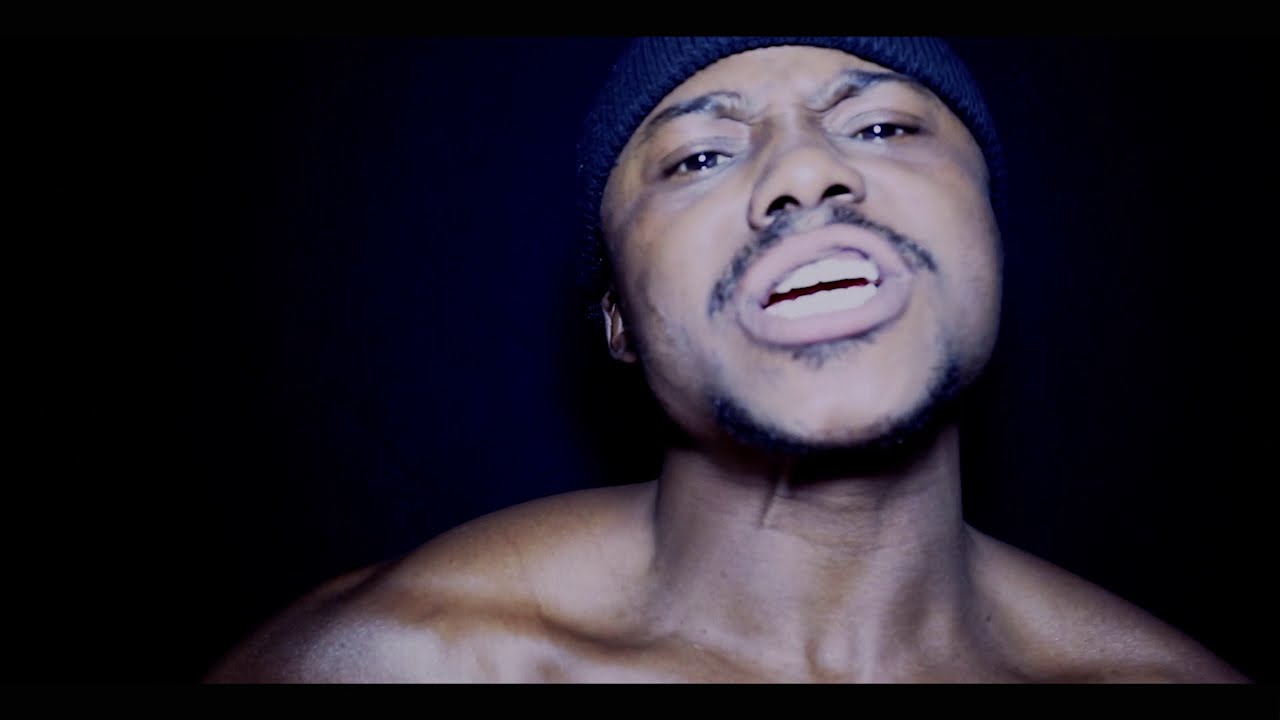This image captures a close-up frame of a black man, possibly in a music video, as he appears to be either singing or rapping. He is shirtless, revealing the outline of his neck muscles and collarbones, with large trapezius muscles suggesting he is fit. He wears a black knit cap and has distinct facial hair: black eyebrows, a black mustache, and a light goatee that frames his chin. His facial expression is intense and focused, with his forehead frowning and his eyes half-closed, conveying a sense of either deep concentration or distress. The background is a very dark black and blue, with a spotlight brightly illuminating his face and torso. Only the outer portion of his left ear is visible, emphasizing the dramatic lighting that highlights his features against the stark, dark backdrop.